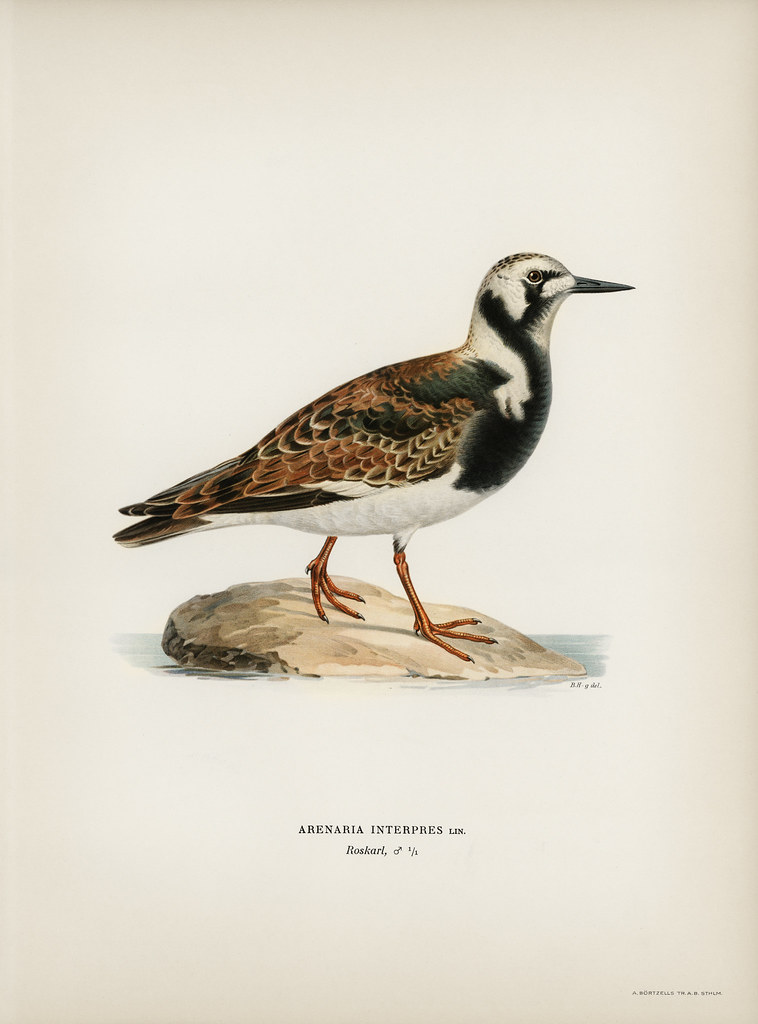This digitally rendered, pencil-style color drawing depicts a bird standing on a rock in a sandy area, likely resembling a beach. The bird is shown in a left-facing side profile, highlighting its sharp, black pointed beak and deep brown eyes. Its plumage showcases a striking combination of white, black, and various shades of brown, including a black breast, a spotted brown crown, and intricate feathering that extends to its tail. The bird's wings are a mix of these colors, adding to its detailed appearance. Perched on the rock, the bird has orange taloned feet with three sharp claws on each. Below the image, the caption reads "Arnaria interpres, L-I-N. Roscarl" and includes the male symbol, signifying its species and sex.